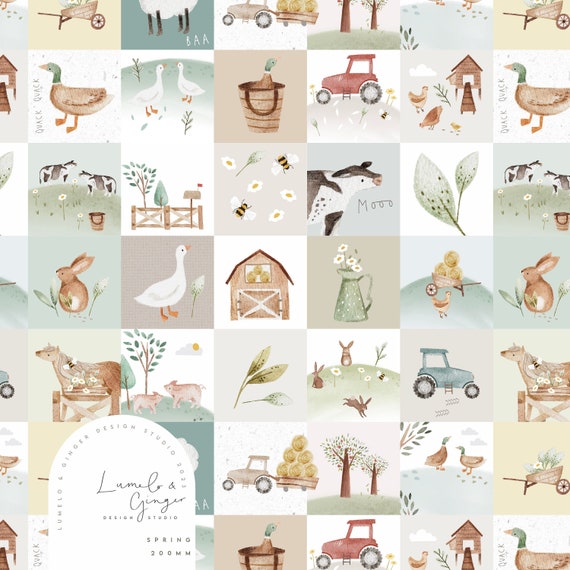This vibrant tablecloth from Lumello and Ginger Design Studio's 2021 Spring Collection showcases an array of charming, rustic illustrations. At the center is a white patch bearing the text "Lumello and Ginger Design Studio 2021," identifying the brand and year. The tablecloth features a series of square blocks, each adorned with different sketches and pictures. One square depicts a single duck, while another shows a pair of white ducks. There is also an image of a bucket filled with a chicken, a red tractor trailer, and a cozily crafted chicken coop where chickens and chicks are depicted pecking at food on the ground. In other blocks, thick green leaves, a grazing cow with the text "moo" beneath it, and a vase brimming with flowers add to the pastoral theme of the design. This collection reflects a blend of farm life and natural beauty, rendered in a delightful, illustrative style.